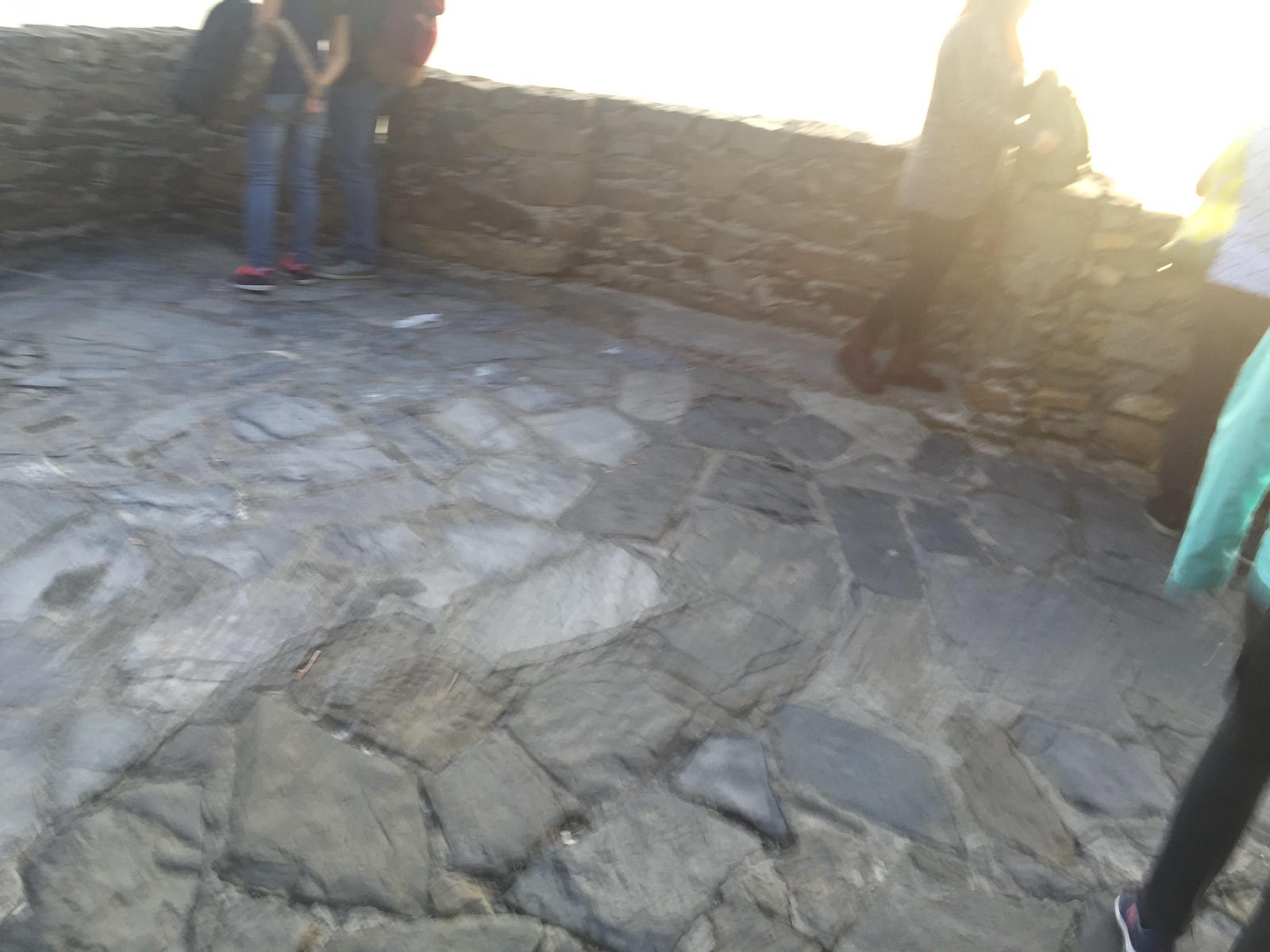This image captures a somewhat blurry and elevated perspective, possibly from the upper portion of a castle or a high balcony, featuring a distinctive rock-tiled floor. The stones vary in colors—gray, black, and bluish—and come in different shapes and sizes, including squares, rectangles, triangles, and circles. The scene shows a small area with a waist-high rock wall, composed of brown stones, over which several people are leaning or standing, suggesting a vantage point with a considerable height. 

There are at least five people visible, although their faces are indistinguishable due to the low angle of the shot. One notable figure, dressed in a turquoise long-sleeve shirt and black pants, possibly sweats, is depicted in fitness or gym shoes. Another individual nearby is seen wearing jeans and a black t-shirt, holding a jacket. To the center, there's a lady carrying a backpack, also in black pants and long sleeves. A man beside her is wearing brown attire, seemingly with his son, distinguished by a short-sleeve white shirt and black pants. Further right, a small person in blue long sleeves and black pants stands by, wearing tennis shoes. A distinct glow or bloom of light is visible off to one side, adding to the ethereal quality of the photograph.